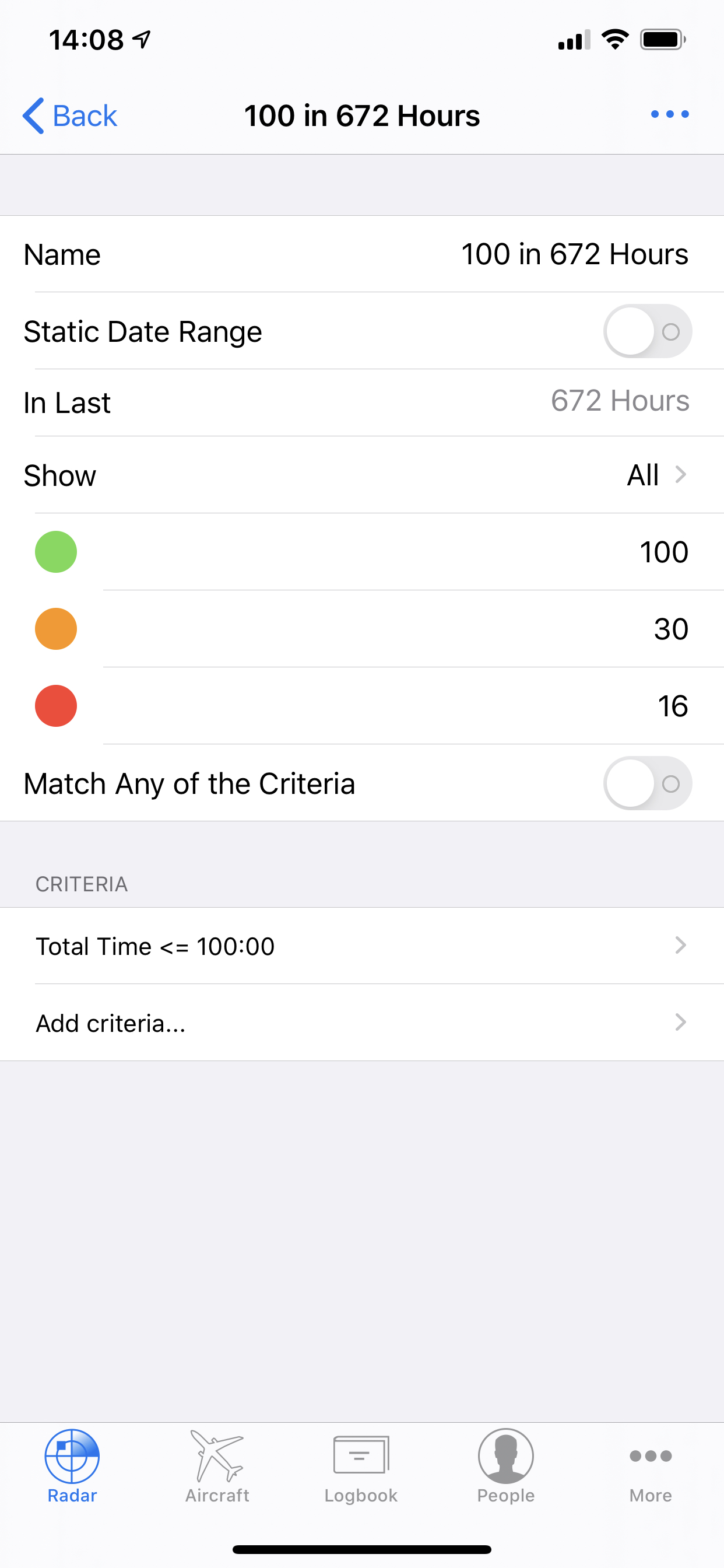This is a detailed screenshot of a mobile phone displaying an aircraft simulation or tracking app. The time on the phone is in military format, showing 14:08. The interface highlights various settings and statistics, `100 in 672 hours` prominently displayed at the top. On the left side, there's a section labeled `Name`, followed by options for `Static Date Range`, `In Last`, and `Show`. 

Three colored indicator dots denote different status levels: the green dot corresponds to `100`, the orange dot to `30`, and the red dot to `16`. 

At the bottom of the screen, a navigation bar features several icons labeled `Radar`, `Aircraft`, `Logbook`, `People`, and `More`. The `Radar` icon stands out in blue, indicating it is the currently selected section, while the other icons are grayed out. 

The detailed layout and specific language indicate that this is likely an aviation-related application, possibly for aircraft tracking or simulation.